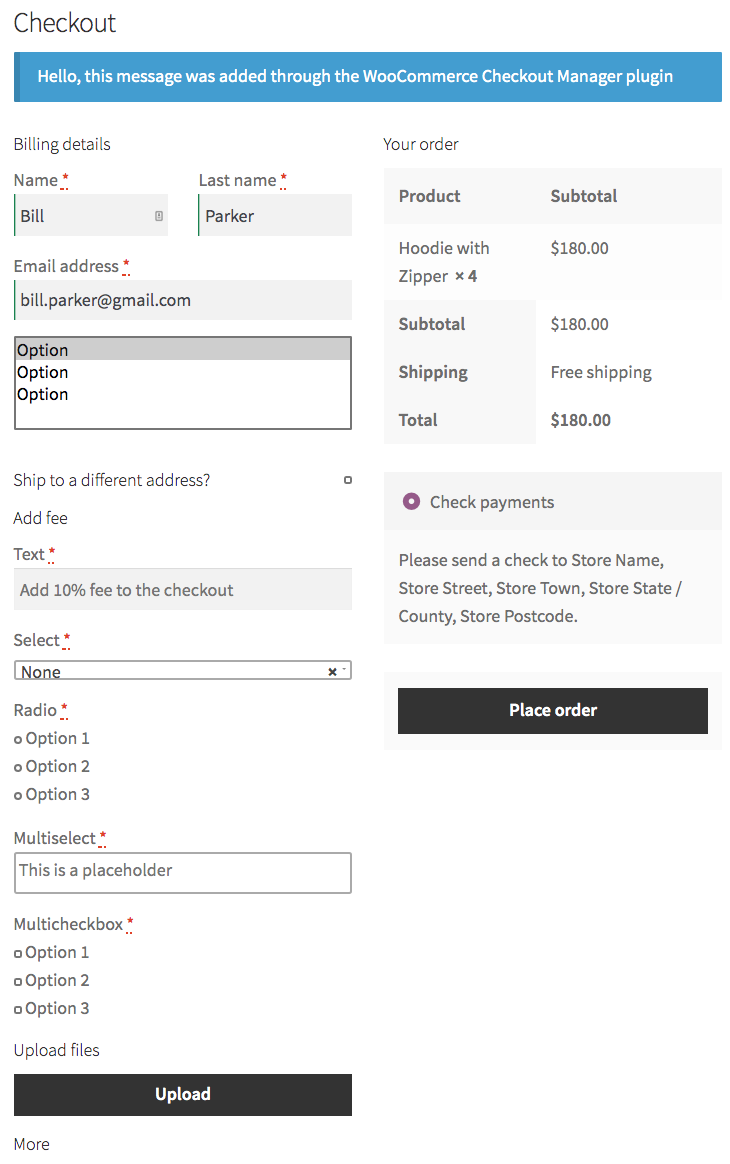**Detailed Website Checkout Page Description:**

This image showcases a website's checkout page, intricately designed for user interaction. 

- **Header:**
  - Positioned at the top left, there is the word "Checkout" written in black letters, serving as a clear indicator of the page’s purpose.

- **Welcome Message:**
  - Below the header, a blue box displays the greeting "Hello" in white letters. This welcoming text is implemented using the WooCommerce Checkout Manager Plugin.

- **Billing Details Section:**
  - The next section is dedicated to "Billing Details," with a prompt to fill in personal information. 
  - **Details:**
    - **Name:** Bill Parker
    - **Email Address:** billparker@gmail.com
  - An options box labeled "option, option, option" is situated below the personal details fields.
  - A checkbox titled "Ship to a different address" is available for users who wish to specify an alternative shipping location.

- **Additional Fields:**
  - Below the aforementioned details, various custom fields include:
    - **Add Fee Text:** Instructions to "add 100% fee to checkout," indicating an additional cost option.
    - **Radio Buttons:** Options listed as "Option One," "Option Two," and "Option Three."
    - **Multi-Set Checkboxes:** Additional choices provided as "Option One," "Option Two," and "Option Three."
    - **File Upload:** A provision to upload files via a black button labeled "Upload" in white letters.

- **Order Summary Section:**
  - To the right of the billing details is the "Your Order" section:
    - **Product Details:** 
      - Product: Hoodie with Zipper priced at $190
    - **Subtotal:** Listed as $180 (appears to be a discrepancy with the product price)
    - **Shipping:** Indicated as free
    - **Total:** Summarized as $180

- **Payment Method:**
  - The "Check Payments" option is marked by a purple circle with a white dot. It instructs customers to "Send a check to" with placeholder text for store name, address, town, state, country, and postcode.

- **Final Step:**
  - At the bottom of the page, there is a prominent black button labeled "Place Order" in white letters, guiding the user to finalize their purchase.

This structured layout aims to facilitate a seamless checkout experience, while incorporating various interactive elements.